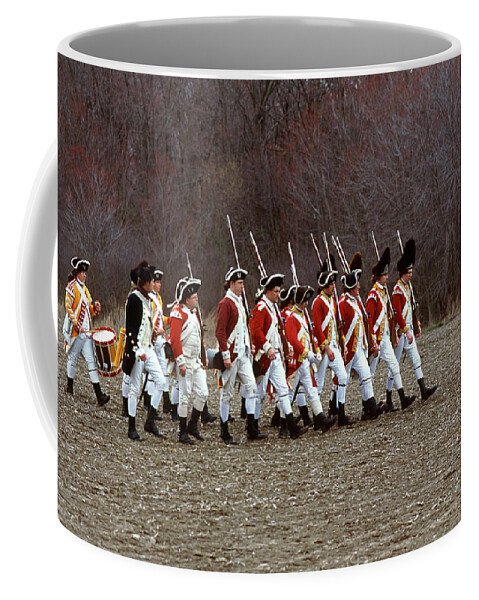In this image, we see a custom-designed coffee mug with a vivid and detailed picture. The mug itself is primarily white, including the handle, interior, and top rim. The printed image on the mug depicts what appears to be a historical reenactment or a scene reminiscent of the Civil War era. The group of around ten soldiers is dressed in distinctive bright red jackets paired with white pants and black boots. Each soldier carries a musket on their shoulder. Notably, there is a figure at the end of the group wearing a yellow jacket, distinct from the rest, who appears to be playing a drum. The soldiers also wear large hats that give an impression of British soldiers. The background of the image is a blurred, grayish forest with dark, leafless trees, providing a stark contrast and highlighting the vividness of the soldiers' uniforms. The scene on the mug captures a lively and historically rich moment, making it a unique and custom piece.